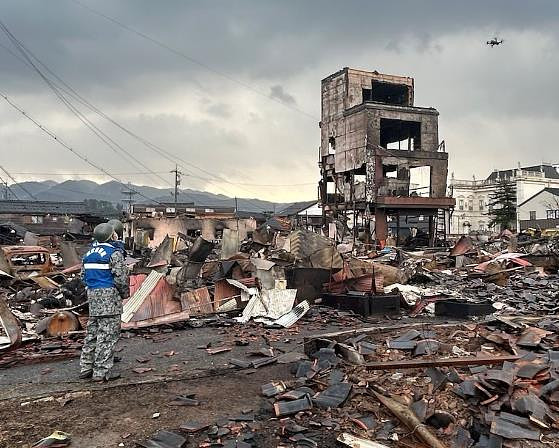The image depicts a desolate scene, likely from a war zone or natural disaster. The sky is filled with dark gray clouds, adding a somber tone to the landscape. In the background to the left, a distant mountain range can be seen, while in the upper right corner, a small plane flies overhead. The foreground is dominated by a man dressed in military attire—camouflage jacket and pants, a bright blue vest, and a dark green helmet. He stands alone amidst the widespread devastation, surrounded by scattered debris and remnants of destroyed buildings. The ground is littered with rubble, and the remaining structures are in various states of collapse. A partially standing building, stripped to its frame with missing walls and windows, stands out prominently. In the background, another intact white building with a gray roof and ornate stonework hints at the area's former state. The scene is chaotic, with debris and destruction everywhere, and no visible writing provides context to the location or events that transpired.